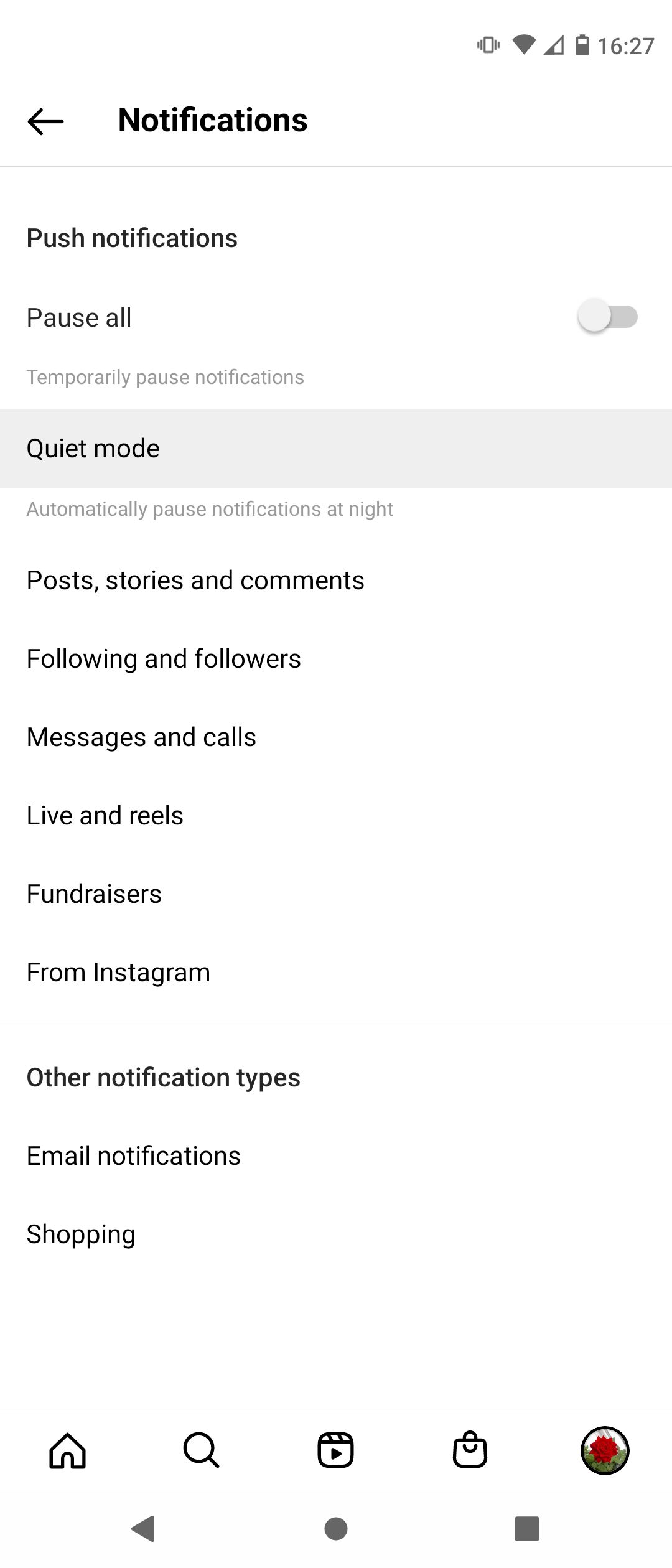The image displays a mobile phone screen showcasing a mobile app's notification settings. At the top of the screen, the status bar indicates the battery level at approximately 50% and the time as 16:27. Directly below, a left-pointing arrow serves as the back button, and in bold, black text, the heading "Notifications" is displayed. Under this, the subheading "Push Notifications" appears.

The first option under "Push Notifications" is "Pause All," accompanied by a toggle switch to enable or disable this feature. Below this is a note in smaller, gray text stating, "Temporarily pause notifications." The next option is "Quiet Mode," with a similar gray-text explanation underneath, "Automatically pause notifications at night."

Following this are a series of specific notification categories: "Posts, Stories, and Comments," "Following and Followers," "Messages and Calls," "Live and Reels," and "Fundraisers." Each category is presented in bold text.

Next comes the "From Instagram" section, followed by "Other Notification Types," "Email Notifications," and "Shopping."

At the bottom of the screen, there's a navigation bar with icons for Home, Search, Video, Shopping, and the User's Profile. Additionally, three more icons—a left arrow, a circle, and a square—are situated beneath this row, presumably for further navigation or functions.